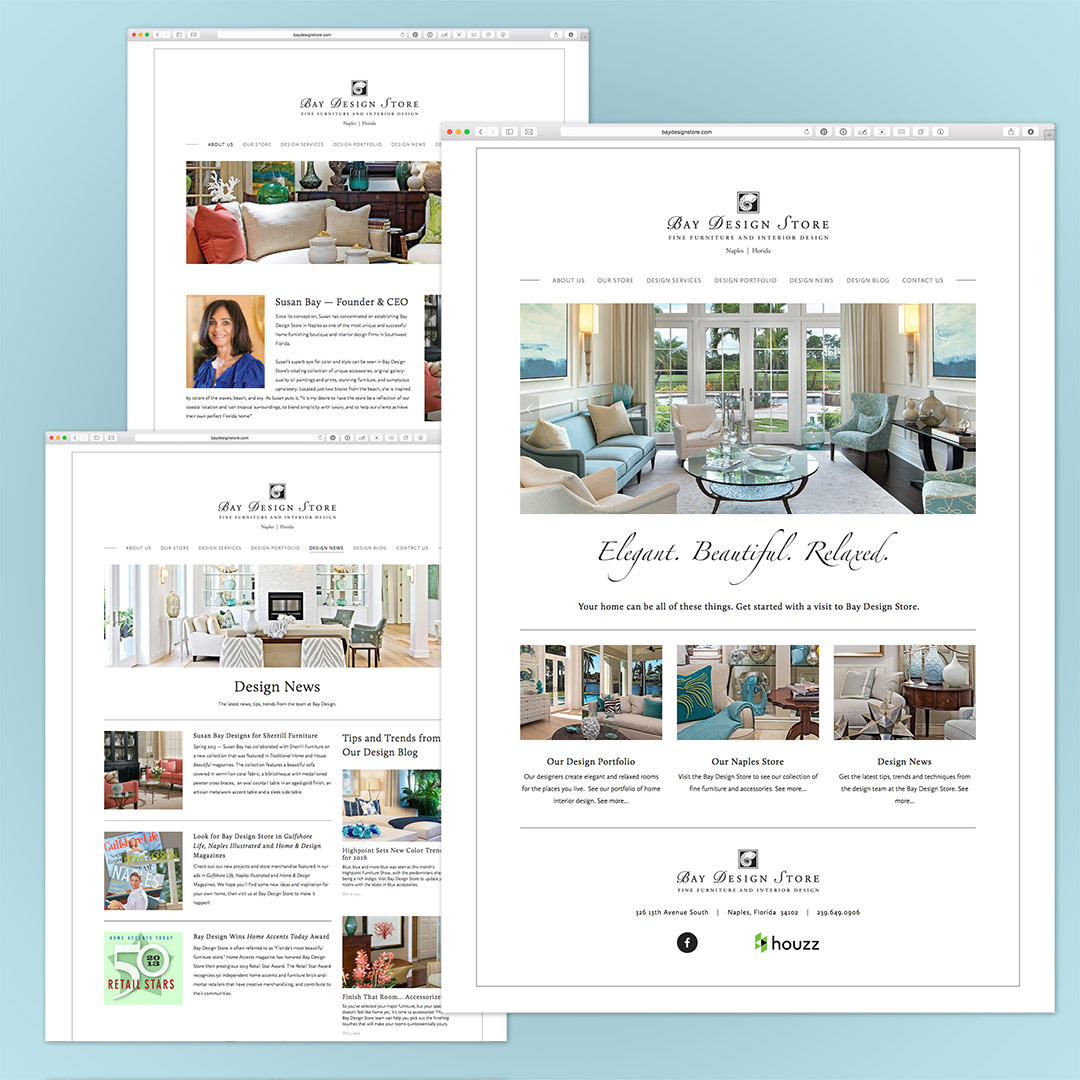The image is a screenshot of a website with a blue background featuring multiple sections showcasing various interior design elements from Bay Design Store. 

On the right-hand side, the top of the section reads "Bay Design Store" and displays an image of a modern living room with large windows opening out to a yard. The room features a green couch on the left, a recycled glass coffee table in the center, and a couple of chairs on the right. Beneath the image, the text reads: "Elegant, beautiful, relaxed. Your home could be all of these things. Get started with a visit to Bay Design Store." Below this promotional text, there are further links labeled "Our Design Portfolio," "Our Naples Store," and "Design News," accompanied by images of other elegant interiors.

The left-hand side showcases another webpage from the same company, featuring a different living room arranged with white couches and greenish chairs against white walls. It is labeled "Design News."

At the top section of the screenshot, there is a close-up image of a white couch adorned with orange throw pillows and a brown desk placed behind it. Adjacent to this, there is a portrait of Susan Bay, the founder and CEO of Bay Design Store. She is depicted with brown hair and a blue shirt, smiling at the camera against a pinkish background.